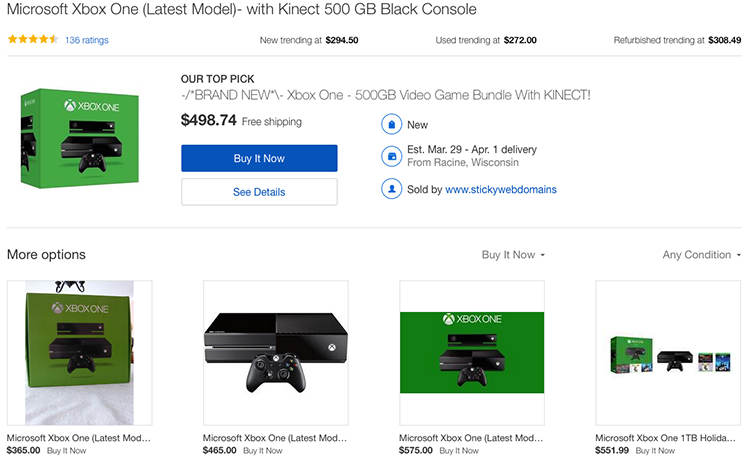This is a detailed screenshot from the Walmart website featuring the Microsoft Xbox One console. The webpage content is cropped, displaying only the search results and product details. At the top left, bold black text reads "Microsoft Xbox One (Latest Model with Kinect 500GB Black Console)." Directly below, a star rating of 5 out of 5 is highlighted, accrued from 136 reviews.

Towards the center bottom, the console's trending prices are listed: 
- New: $294.50 
- Used: $272.00 
- Refurbished: $308.49

Directly beneath this information, there's a label indicating "Our Top Pick." The featured item is a brand new Xbox One 500GB Video Game Bundle with Kinect, priced at $498.74, inclusive of free shipping (noted in small gray text). Below this, a prominent blue "Buy It Now" button is displayed, followed by a blue outlined "See Details" bar.

To the right of these buttons, there are three icons:
1. A sales tag icon labeled "New."
2. A box icon with a delivery estimate of March 29th to April 1st, noted to ship from Racine, Wisconsin.
3. A profile icon indicating the seller, Sticky Web Domains, a third-party vendor.

Underneath the primary product information, there's a section titled "More Options" on the left, featuring four thumbnails showcasing different sellers and Xbox listings.